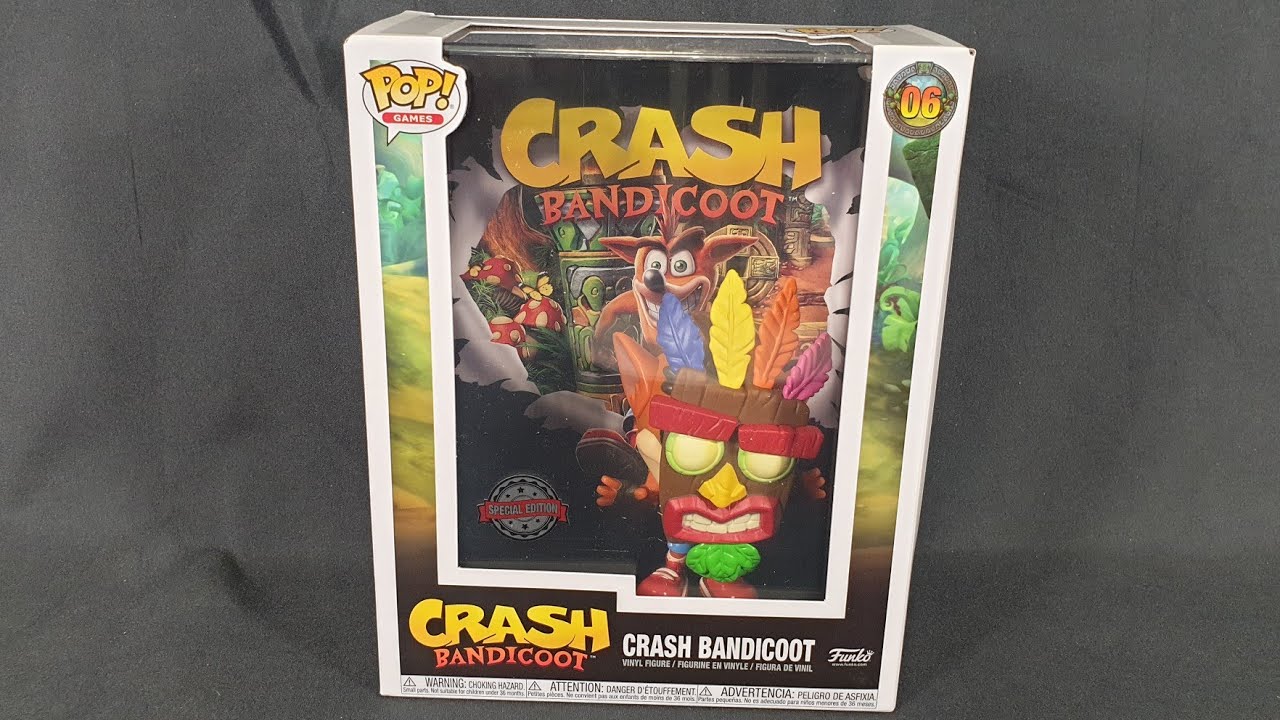The image depicts a boxed Funko Pop figure from the video game series Crash Bandicoot. The packaging is rectangular and primarily white, featuring a large plastic window offset to the right, through which the figure is visible. In the upper left corner of the box, "Pop!" is written in yellow with an exclamation mark, followed by "Games" in red text. In the upper right corner, inside a circle, is the number 06. The name "Crash Bandicoot" is prominently displayed in large yellow letters for "Crash," and smaller orange or red letters for "Bandicoot."

The Funko Pop figure itself appears to be a stylized version of a character from the game, featuring a brown, big-eyed, large-nosed figure with a big grin. Below this character, another distinctive figure is visible, resembling a tiki mask made of wooden planks. This character has big, fluffy red eyebrows, glowing greenish-yellow eyes, a red nose, large wooden red lips with white teeth, and a green leaf beneath its mouth resembling a soul patch. Atop its head are four colorful feathers. The character is also depicted wearing blue pants and large, reddish clown-like shoes.